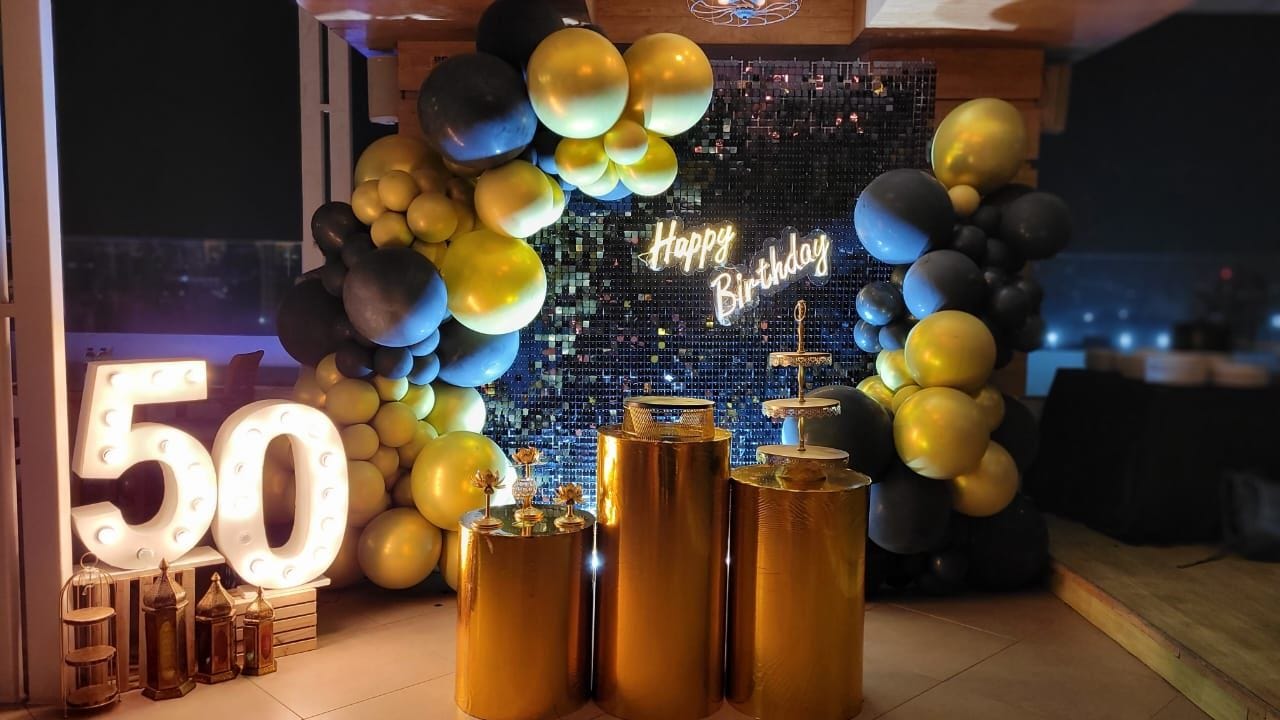In this detailed photograph of an upscale indoor setting, likely an apartment, penthouse, or rooftop bar, we see an elaborately decorated 50th birthday party setup. Dominating the center is a striking neon sign in light yellow that reads "Happy Birthday," mounted on a glittering wall made of reflective pieces. Flanking this central feature are two balloon arrangements; the left forms an arch that curves overhead, while the right stands vertically. The balloons themselves are a mix of large and small sizes in gold and navy blue hues.

To the left of the neon sign, wooden blocks support large illuminated numbers "5" and "0" at varying heights, indicating the milestone birthday. Front and center in the image stand three golden podiums of differing heights. The leftmost podium holds what appears to be golden drink glasses, the central one has a shiny, reflective tin, and the rightmost podium features an empty, three-tiered cake stand.

In the background to the right, the setting transitions onto a wooden platform, where a table adorned with a dark black tablecloth displays neatly stacked white crockery plates. The overall decor suggests a sophisticated and meticulously planned celebration, blending sparkle, illumination, and luxurious touches.